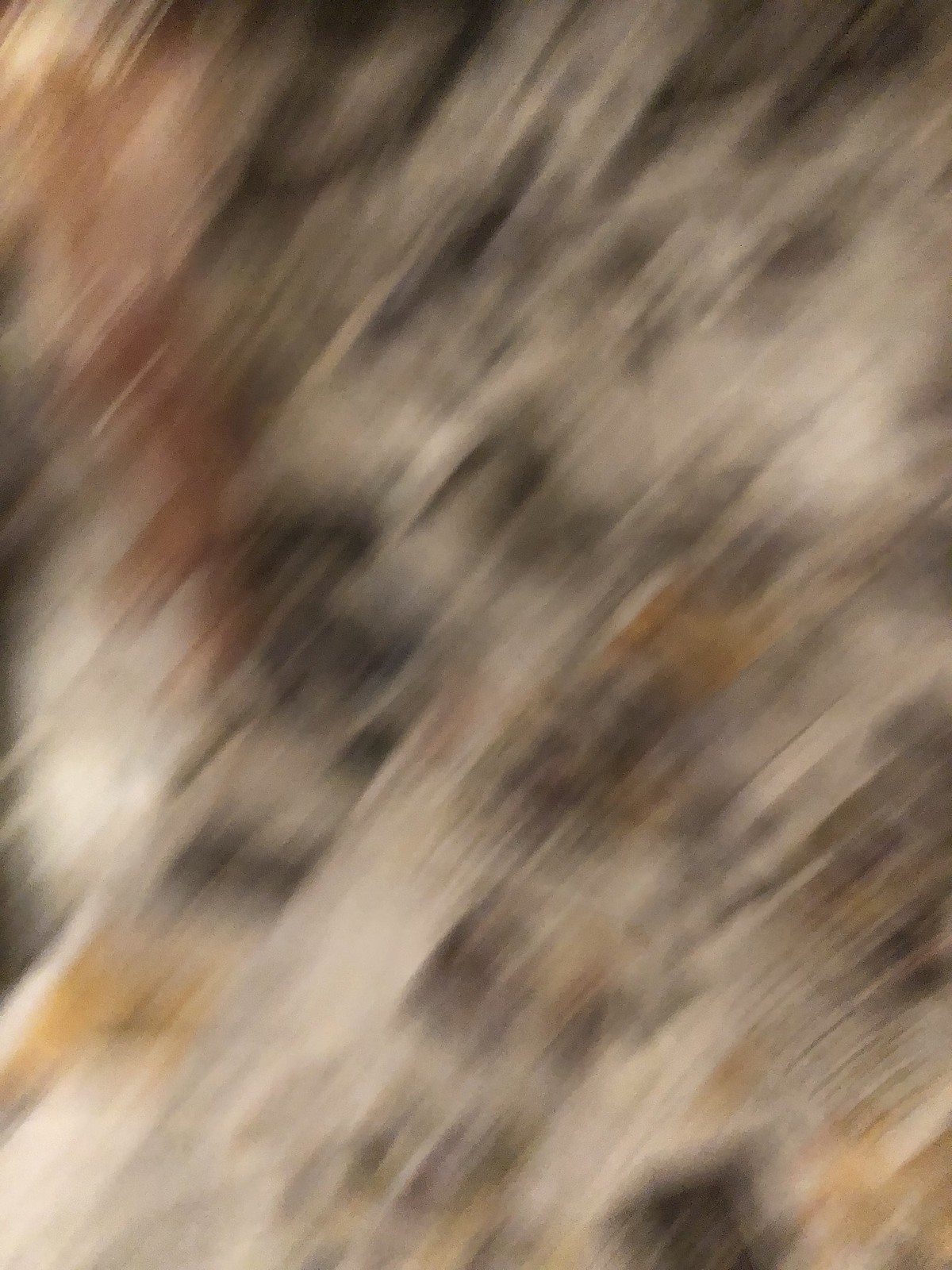A vibrant abstract artwork dominates the frame, characterized by dynamic diagonal strokes that stretch from the bottom left to the top right. The composition is a riot of colors, with bold white lines intersecting splashes of black, red, orange, yellow, and gray. The brushstrokes create a sense of energetic motion, resembling chaotic scratches across the surface. The image is intentionally blurred, adding to its abstract nature and leaving the subject open to interpretation. This expressive piece defies clear identification, evoking a sense of unrestrained creativity and artistic freedom.